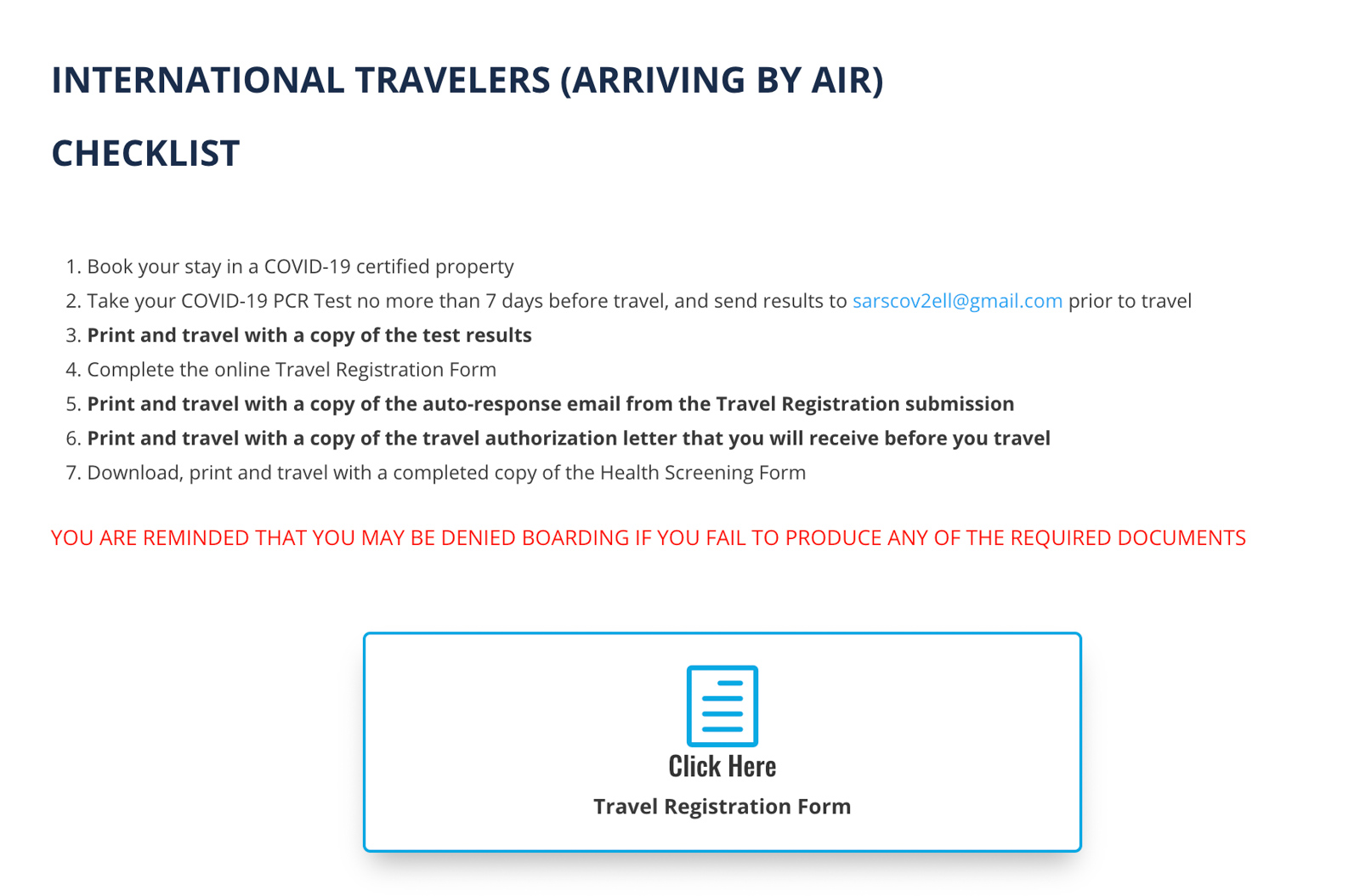The image captures a page from a digital device displaying a checklist for international travelers arriving by air. The title at the top reads "International Travelers" with a subtitle in parentheses stating "Arriving by Air Checklist." Below the title, there are seven items listed consecutively in a vertical arrangement on the left side. 

1. The first item advises travelers to book their stay in a COVID-19 certified property.
2. The second item instructs travelers to take a COVID-19 PCR test no more than seven days before travel and to send results to SARSCOV2ELL at gmail.com prior to travel.
3. The third item, which is highlighted in bold, advises travelers to print and travel with a copy of their test results.
4. The fourth item requires travelers to complete the online travel registration form.
5. The fifth item states that travelers should print and travel with a copy of the auto-response email received after submitting the travel registration form.
6. The sixth item, also in bold, emphasizes the need to print and travel with a copy of the travel authorization letter that will be received pre-travel.
7. The seventh item instructs travelers to download, print, and travel with a completed copy of the health screening form.

At the bottom of the checklist, in red text, there is a reminder that travelers may be denied boarding if they fail to produce any of the required documents. Finally, there is a blue rectangle with the link "Click here Travel Registration Form."